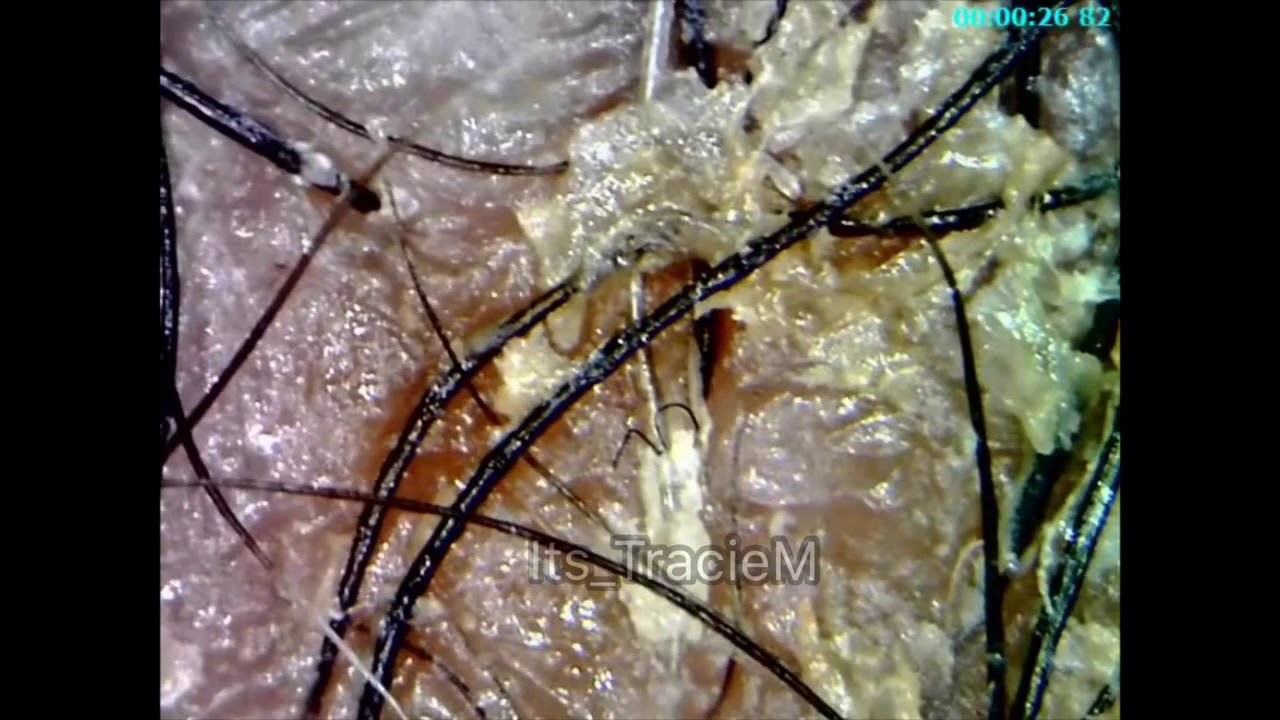The image is an extreme close-up, revealing a highly detailed and somewhat unsettling view that seems to depict human skin with black hair follicles. There's a gelatinous substance, likely mucus or pus, prominently visible at the top right and towards the center. The left side of the image displays a pink hue, transitioning to yellow in the middle and green on the right. Scattered throughout are black strands resembling both fine hairs and thicker twigs, crisscrossing in various directions. Among these, two particularly fine black hairs create a loop shape. A blue timestamp is partially visible in the top right corner, reading "2682." At the very bottom center in a white, semi-transparent watermark, the text "Its Tracy M" is clearly displayed, with "T" and "M" in uppercase and the rest in lowercase. The overall composition and color palette of the image—along with the mixed textures and elements—create a visually striking, but not appetizing, scene.